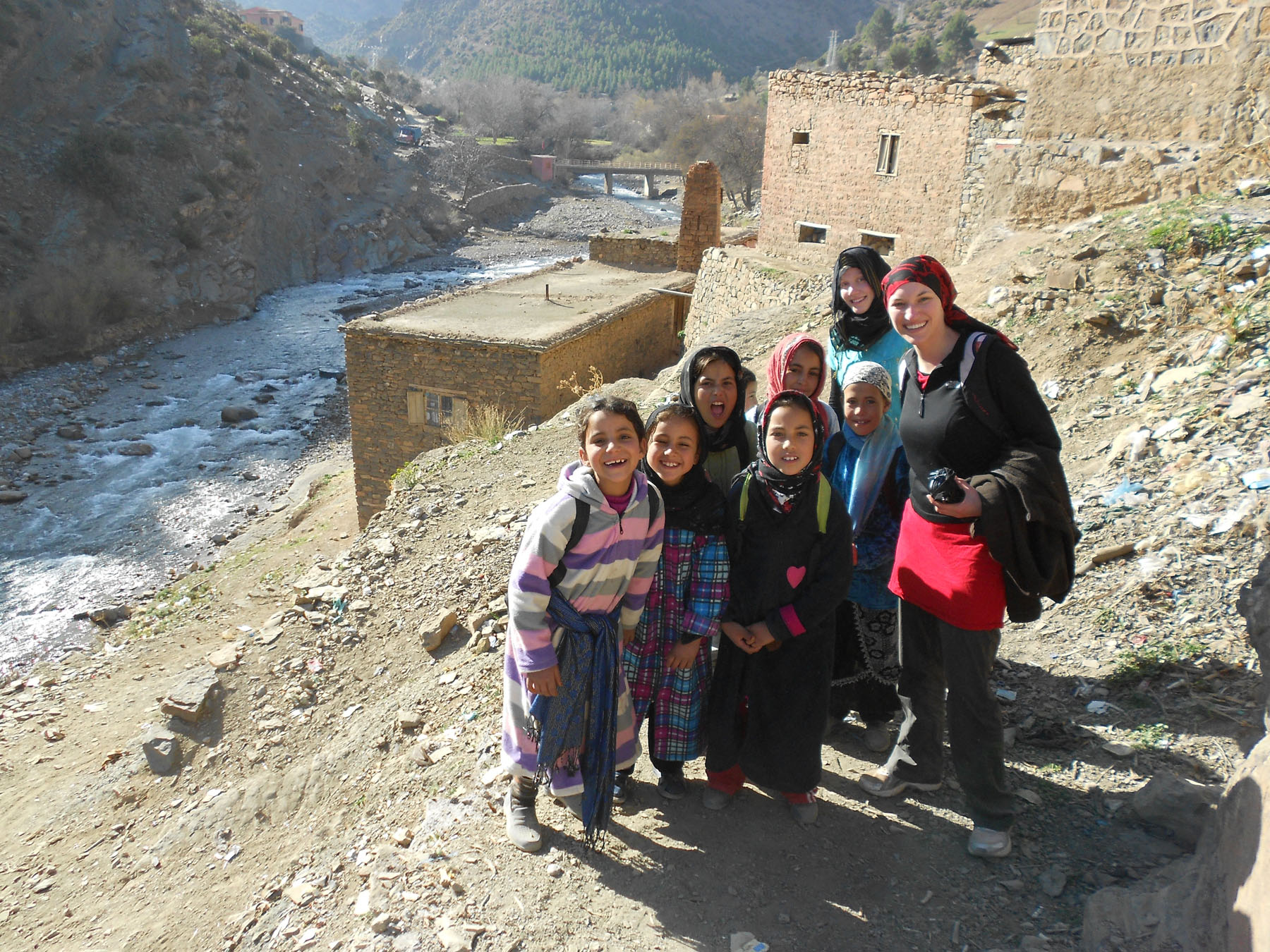In the photograph, a group of eight individuals—two women and six children—pose on a gravelly hilltop in what appears to be a region such as Iraq, Iran, or Afghanistan. The women and the majority of the children, who seem to be predominantly female and around ten years old, are wearing traditional Muslim hijabs. The woman in the forefront, smiling warmly, dons a black top, a coral red skirt and pants, and a jacket draped over her arm, her headscarf a striking red and black. The woman behind her is attired in a blue top with a darker colored hijab. The background features a flowing river to the left, framed by rugged mountains. In the distant center, a bridge spans a gully with a visible waterway, and behind the group are old, run-down stone and brick buildings. The scene is painted in earthy tones of brown and beige, with sparse greenery from a few trees dotting the landscape, contributing to the overall desolate yet captivating atmosphere.